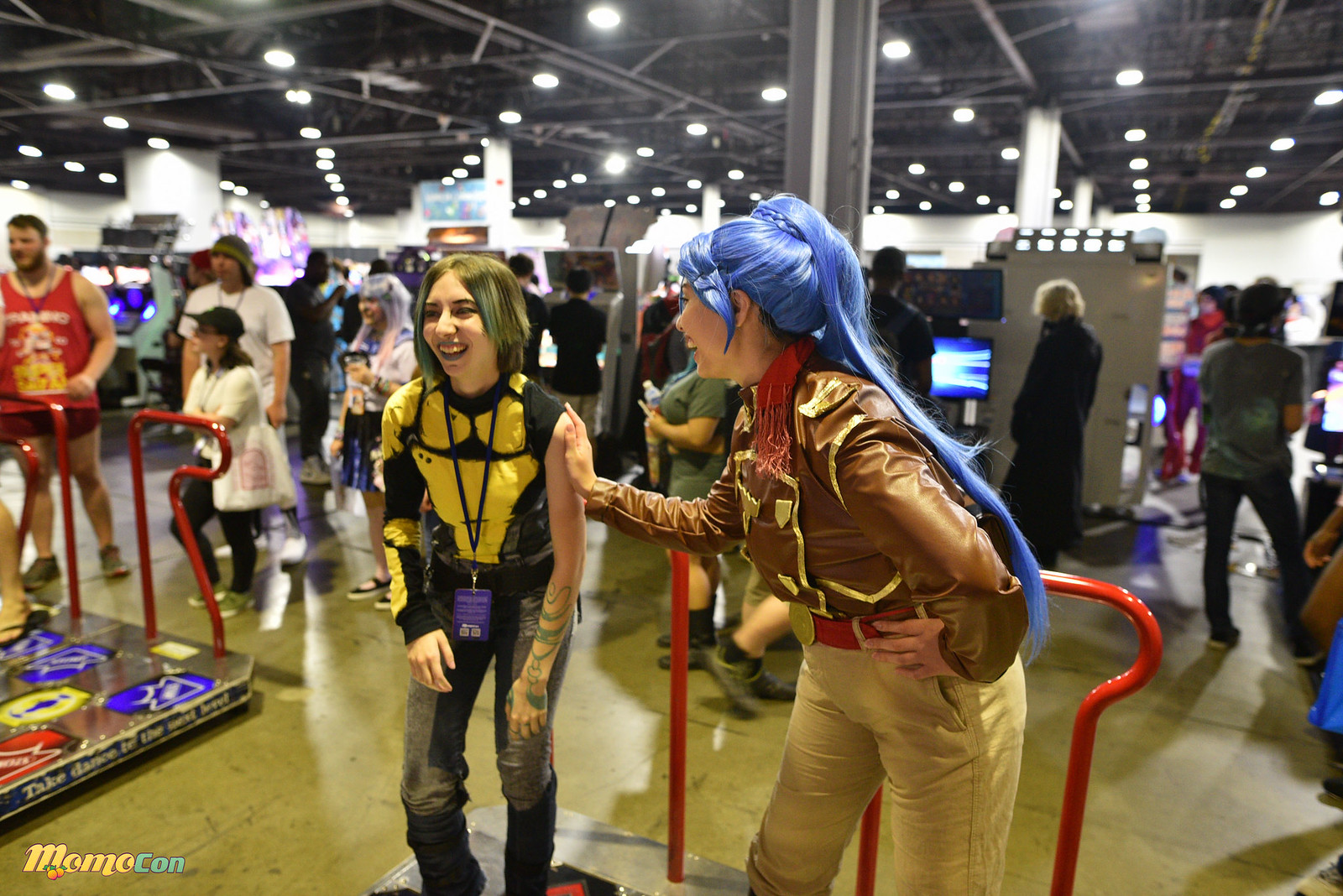The image captures a vibrant cosplay convention inside an expansive convention center, bustling with activity. Two young women are centered on a silver platform, engaged in a lively moment, possibly playing a Dance Dance Revolution-type arcade game. The woman on the left, with short green hair and light skin, is sporting a striking black and yellow one-sleeved top, paired with gray pants. She has a lanyard around her neck and tattoos visible on the lower part of her left arm. The girl to her right is laughing, wearing khaki pants and a distinct brown shirt with gold lining. She dons a long blue wig fashioned into an extended ponytail. Behind them, the expansive space is filled with numerous people exploring various exhibits and games, including another red-bannistered platform to the left. The floor beneath them is a greenish-brown hue, contrasting with the tall black metal ceiling overhead, which is adorned with a multitude of white and yellow lights. To the far left, a man in a red and yellow shirt and red shorts stands before yet another interactive game. The words "manjo.con" are inscribed in the lower corner of the picture, further emphasizing the lively convention setting.